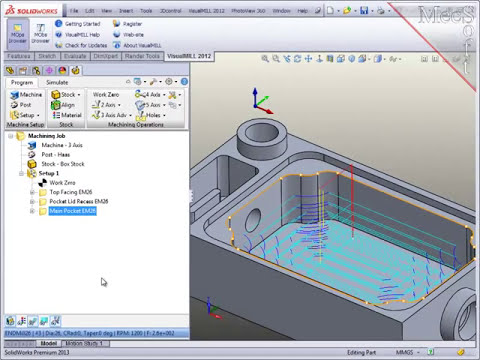The image is a screenshot of a computer monitor displaying the SolidWorks interface. The top left corner prominently features the name "SOLIDWORKS" in red print. Just below the software's name, various command icons are visible, including file, edit, view, insert, tools, and others. A watermark in the top right corner reads "Macsoft". The screenshot also shows a section on the left side with multiple icons labeled as machine, stock, post, setup, material, and align. Beneath these icons, there is a file folder named "MachiningJob" containing numerous files.

On the right side of the interface, there is a detailed, computer-drawn image of a machine that appears rectangular in structure. This image includes a sink on the right side, a smaller container on the bottom left, and a circular hole in the top left corner. The machine illustration also features color-coded arrows - blue pointing up, green pointing to the upper right, and red pointing to the lower right - which likely indicate different axes or movement directions. The machine's design has gray tones with hints of green and blue, possibly representing water within the sink structure.